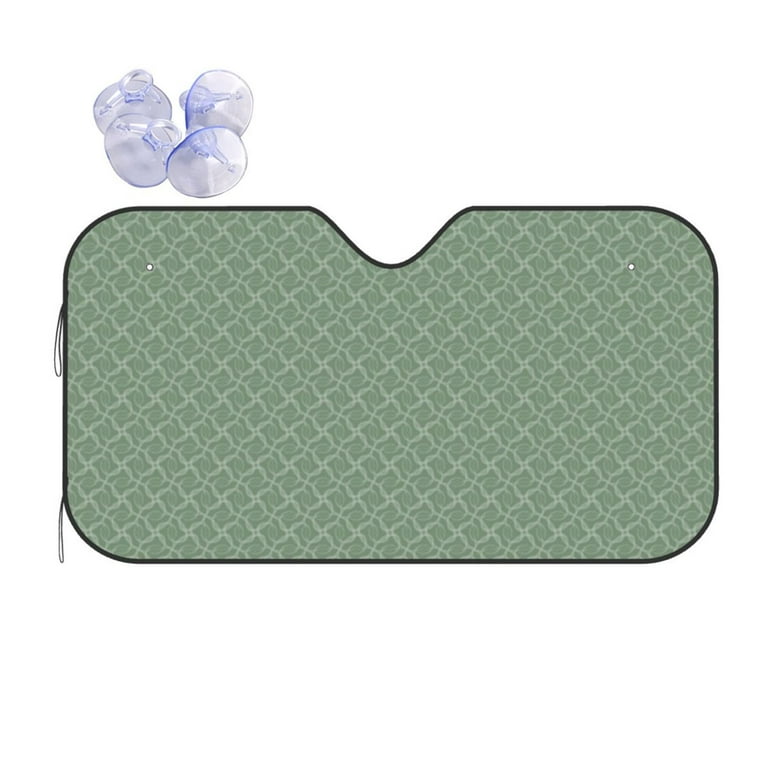This product photograph features a rectangular mat, predominantly dark green with a thin black border. The mat is approximately twice as wide as it is tall, marked by a unique notch at the top that resembles a nose cutout, giving it a subtle geometric flair. The textured surface boasts a patterned design of light green V-shapes forming a loose grid across the jade green background. Two small holes are positioned near the top corners, possibly for the attachment of the four clear rubber suction cups visible in the image's upper left corner. These suction cups feature round parts on the opposite side, presumably designed for secure attachment to a flat surface. Additionally, two black strings extend from the left side of the mat, suggesting another potential mode of securing it. While the precise function of this mat remains unspecified, the detailed design elements indicate a thoughtfully crafted product, potentially a shade, visor, or other utility mat.